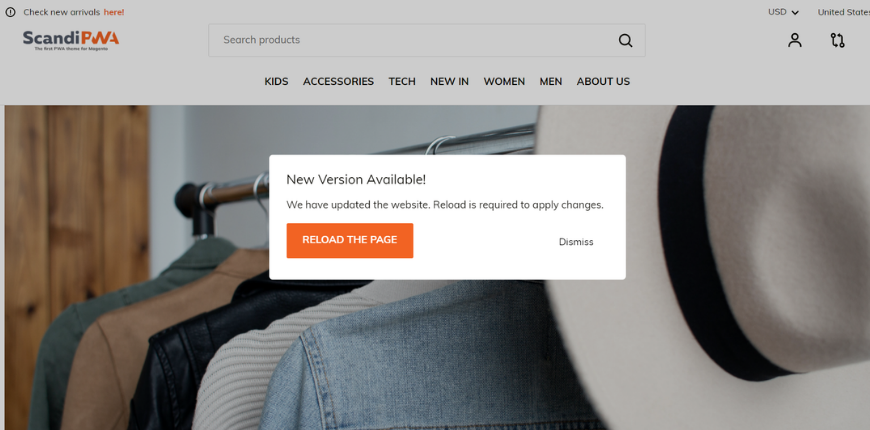The website features a grey navigation bar across the top. On the upper left side, the name "SCANDI" is displayed in black text, followed by "PWA" in large orange letters. Above these, in small print, is the phrase "Check new arrivals here." Centrally positioned on the grey bar is a search button. 

Below the navigation bar, there are several columns labeled "Kids," "Accessories," "Tech," "New In," "Women," "Men," and "About Us." 

In the center of the page, an image displays a clothing rack featuring various jackets. The visible pieces include a grey jacket, a brown jacket, a black jacket, a white sweater, and a blue jean jacket. In the foreground on the right side, a white hat with a black rim is prominently displayed. The background consists of a white wall and, on the left-hand side, a wooden wall with a medium wood finish and noticeable knots.

Dominating the central part of the image is a white notification box with the message: "New version available. We have updated the website; a reload is required to apply changes." Below this text is an orange button labeled "Reload the page" in white letters.